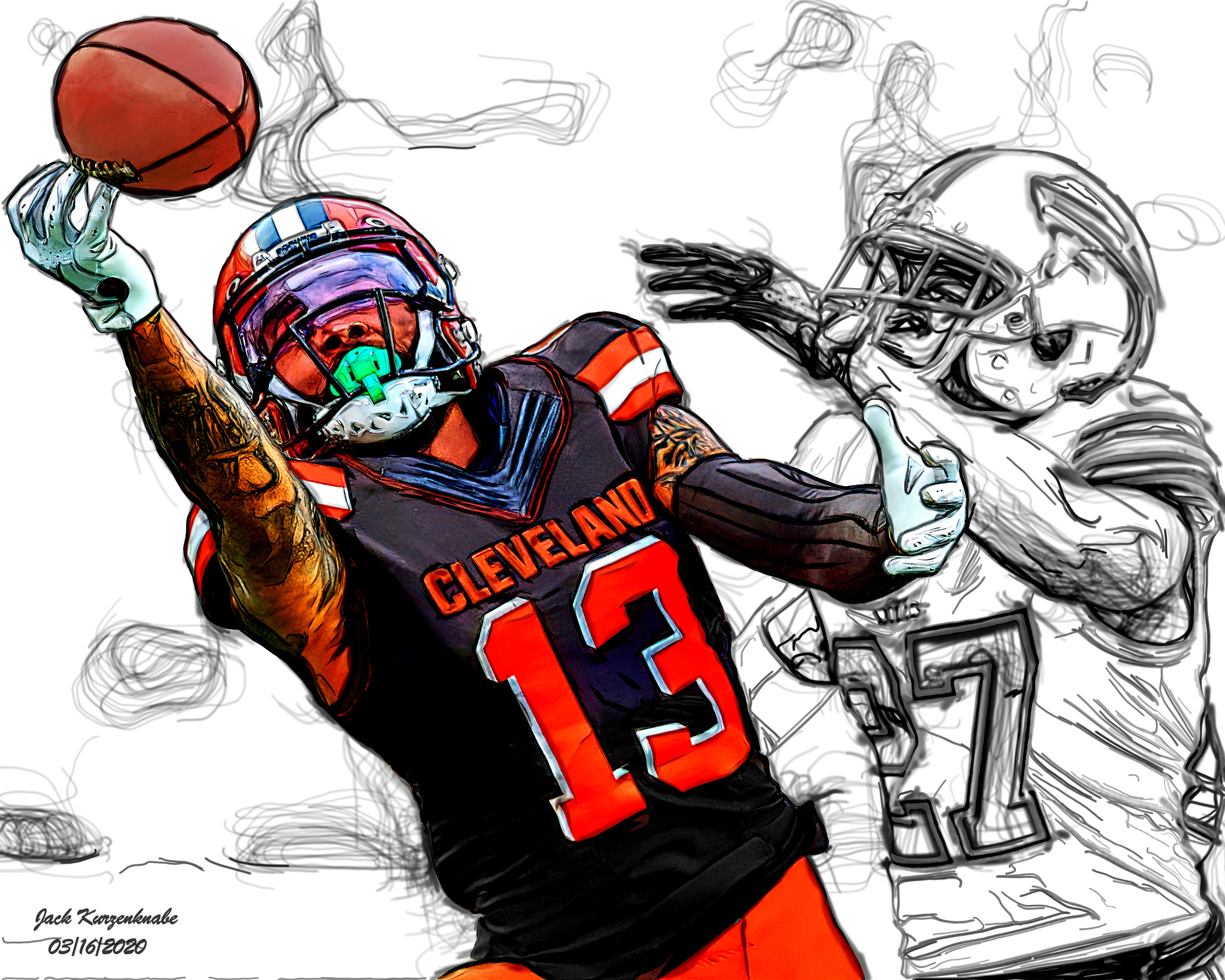This digital illustration vividly depicts a football scene with two players in action. Dominating the left side, a fully colored player wearing a Cleveland Browns jersey with the number 13 is reaching up to catch a football. This player, who appears to be a black man, is adorned with tattoos on his arms, and is equipped with white gloves, an orange helmet, and a green mouthpiece. His navy, orange, and white jersey prominently displays "Cleveland" in deep orange letters.

In contrast, the player on the right side is represented in a sketchy, black-and-white style. This player, who wears the number 27, is in the act of trying to block or tackle and is surrounded by dynamic lines emanating from his head, adding to the illustration's energetic feel.

The background features scribble-like marks, enhancing the contrast between the meticulously colored player and the sketchier, monochromatic one. At the bottom left of the image, the artist's name, "Jack Curson," along with a date, "3-16-2020," are inscribed.